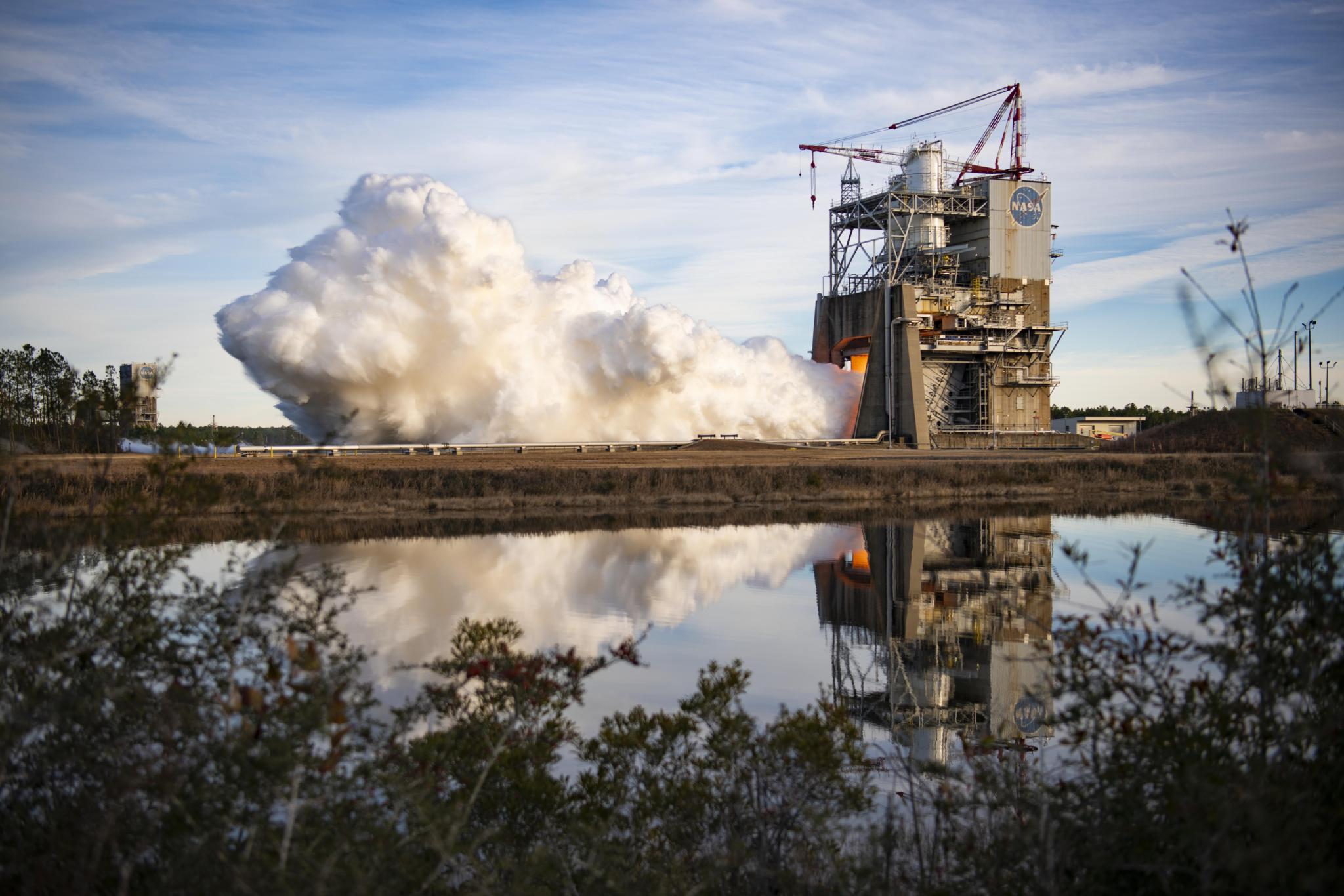This detailed photograph captures a NASA rocket launch pad situated beside a perfectly squared-off water body. The scene is set with blue skies adorned with thin clouds and is viewed from across the lake, where the tops of bushes are visible in the immediate foreground. The land around the facility appears meticulously sectioned into geometric squares. Dominating the image is a robust, industrial building marked with NASA's iconic blue circle emblem and white letters. From this brown, two or three-story structure, a massive plume of white smoke and steam is emitted through an open, large door on the side, suggesting active rocket launch activity. The smoke and the building itself are vividly reflected in the serene water body adjacent to the facility. In the background, a bridge and multiple trees are visible, adding to the composite industrial and natural landscape. A crane is also noted on the platform, further emphasizing the launch preparations. This captivating scene encapsulates the grandeur and meticulousness of a NASA rocket launch setup.